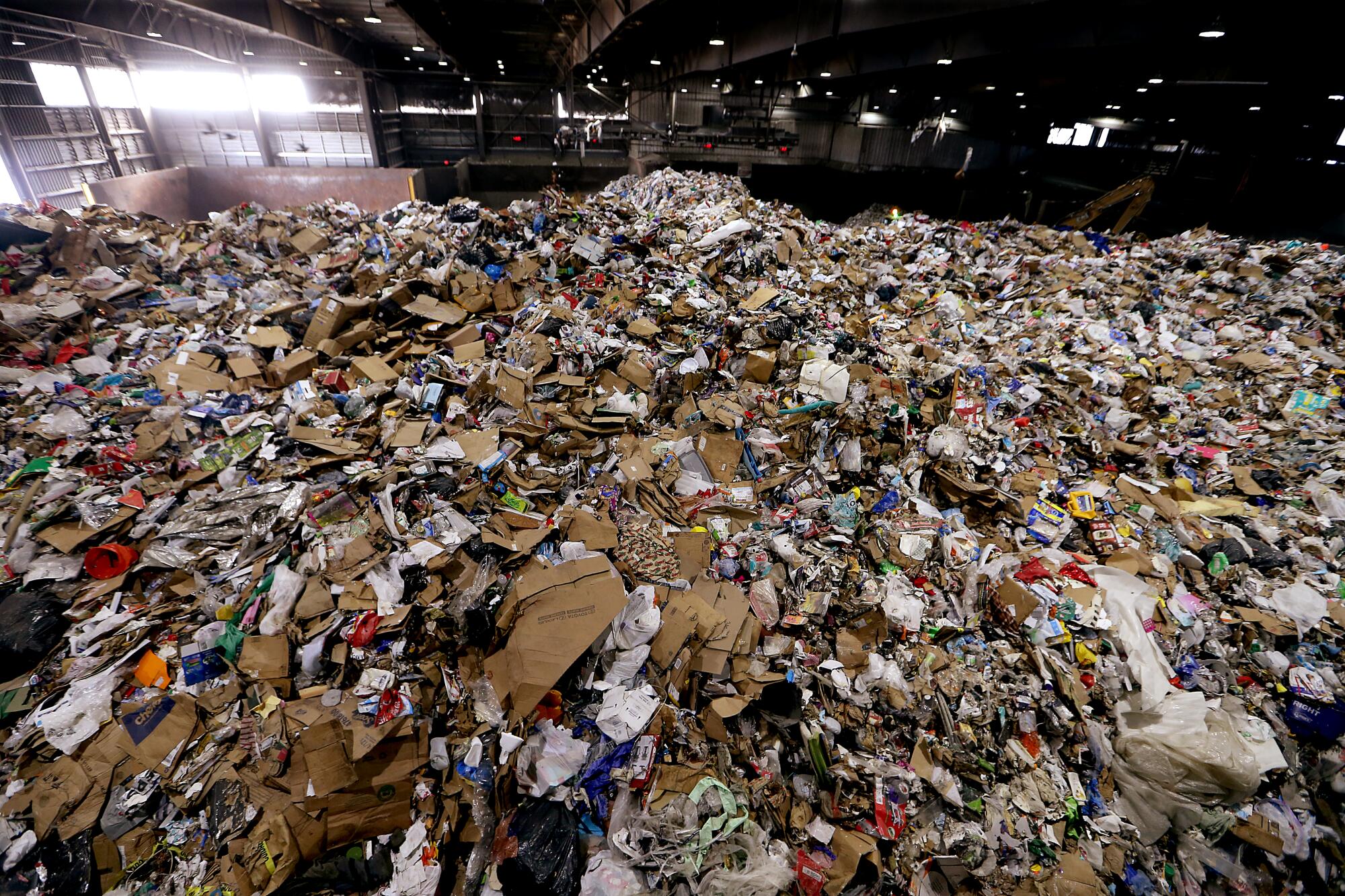The image depicts an indoor recycling plant filled with a substantial pile of recyclables, primarily composed of smashed and flattened cardboard boxes, along with various plastic materials. Dominating the lower three-quarters of the image, the pile includes white, tan, and blue cardboard, with a red bucket and thick commercial white plastic visible towards the bottom. The scene is set in a large warehouse characterized by cement block walls and heavy machinery equipped with arms and scoops, positioned to manage the recycling materials. Sunlight streams through a large window in the top-left corner, while additional lighting fixtures are suspended from the ceiling, illuminating the workspace further. The majority of the materials appear to have been meticulously sorted, devoid of food waste, emphasizing a systematic recycling operation.